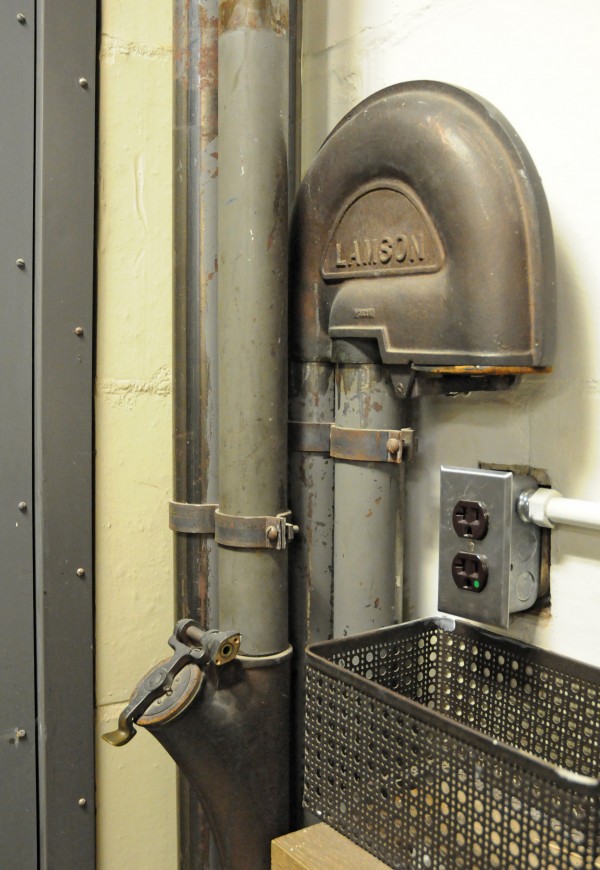In a grungy, industrial-looking corner of a room, an eye-level photograph captures a scene reminiscent of a building's back maintenance area, possibly a basement furnace or water heater space. Dominating the image is a metal pipe that ascends upward in the corner, bolted securely to the white wall. The pipe features a valve or port with a lid that can open, positioned at about waist height and pointing at a 45-degree angle. Above the pipe and slightly higher than the lid is an electrical socket encased in brown plastic. Below the socket, a metal wire basket sits on a table that is largely out of frame. 

On the left side of the image, there's a bolted metal door frame without the door itself visible. Additionally, the metal pipe connects to multiple tubes. Two tubes lead to a rounded metal cap inscribed with the name "LAMSON," while the other two tubes are closer to the wall. The photo also highlights the contrasting colors of grimy white and mildewy yellow walls, enhancing the industrial and neglected atmosphere of the setting.